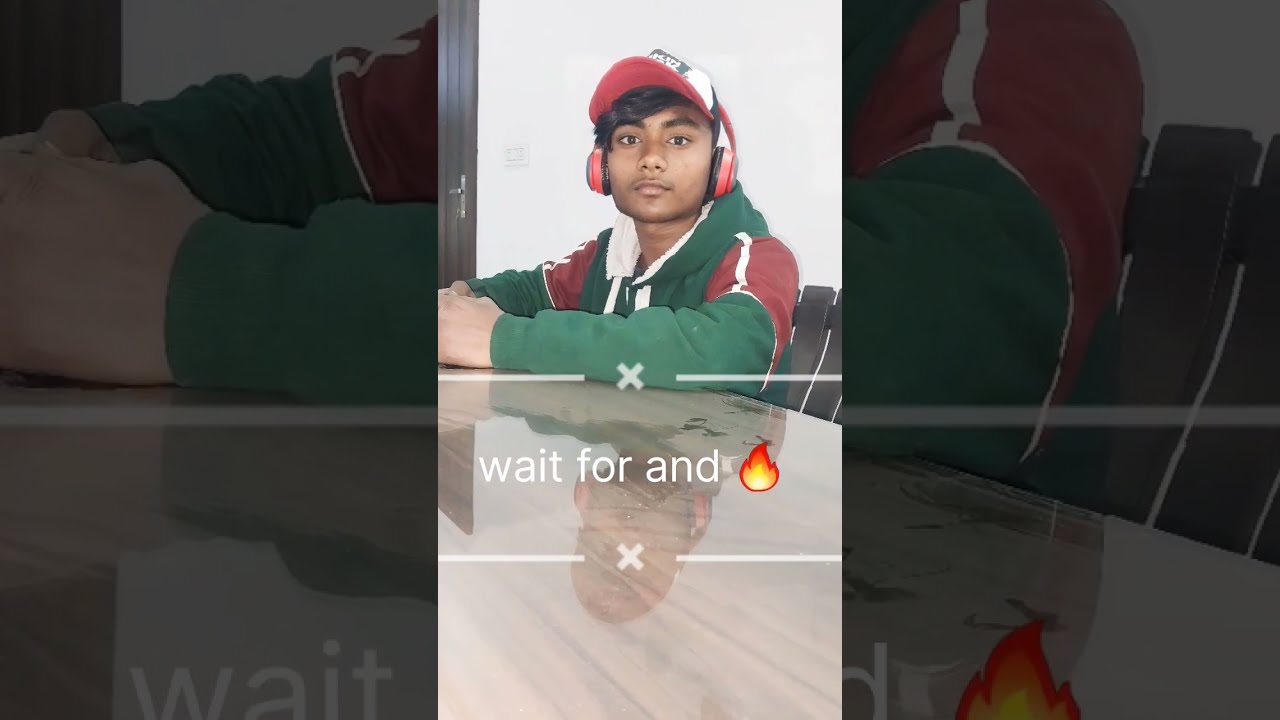The image features a young man, possibly Indian, seated at a glossy, wooden table that has a glass layer on top. He is wearing a baseball cap with a red brim and a white front, and has long black hair peeking out from underneath. He also has red headphones with black foam pads on his ears. His hoodie is predominantly green with red and white-striped biceps, and it also has white drawstrings and a white-lined hood. The man is sitting in a dark brown chair with vertical slats resembling a picket fence, and you can see his reflection on the shiny table surface.

The composition of the image is unique, divided into three sections. The central portion, taking up one-third of the image, prominently features the man. On either side of this central image, the background reiterates the same image but with a black, transparent filter. The left side focuses on a close-up of his hands and arms, while the right side shows a close-up of his upper left arm and part of the chair. The text "wait for" accompanied by a fire emoji is positioned between two white lines with white Xs in the center of each line, spanning across the middle section of the image.